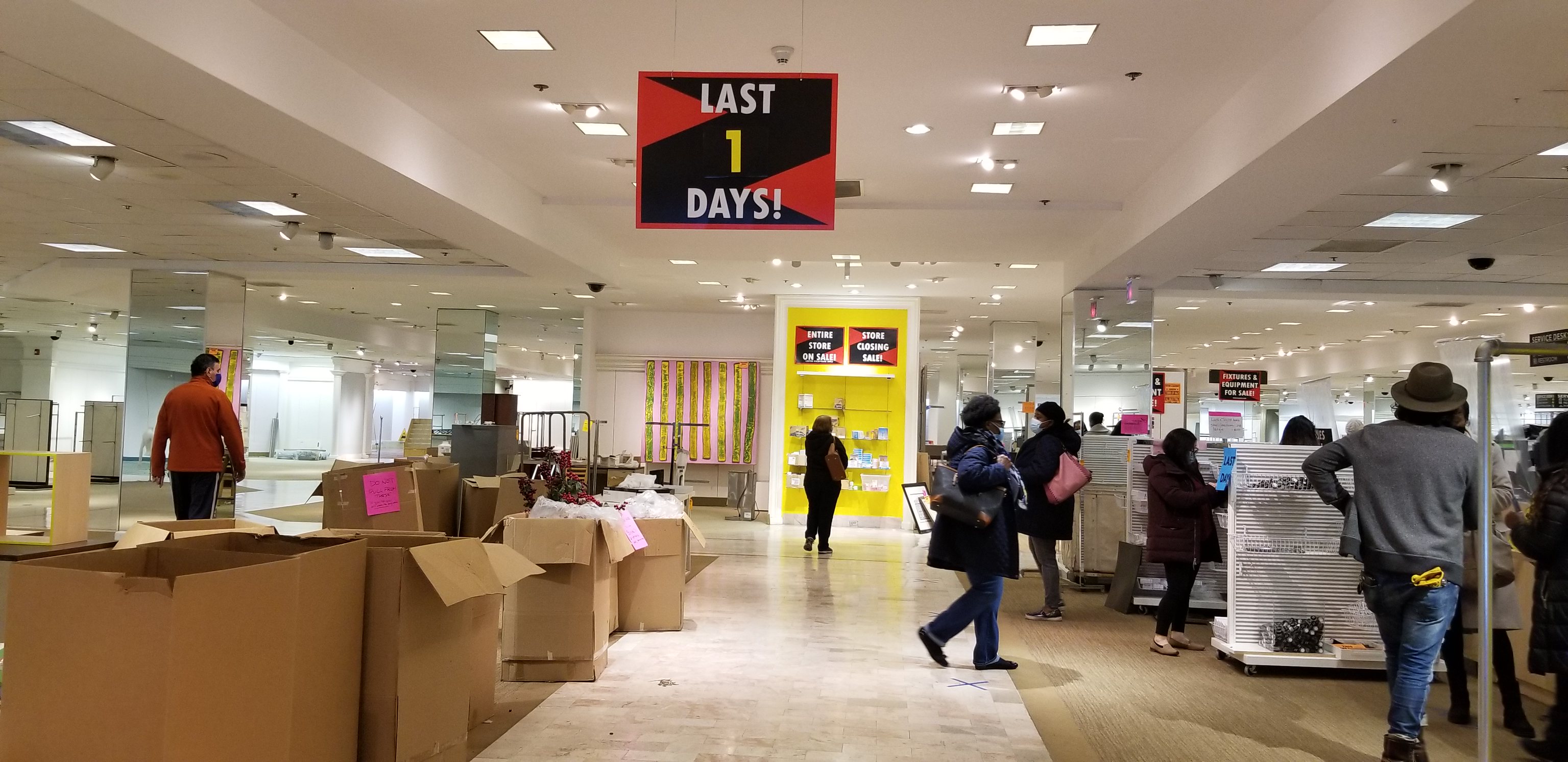The photograph captures the inside of a mostly empty store that is in the process of closing down. The store features white ceilings with square fluorescent lights and mirrored pillars reflecting the sparse interior. In the background, white walls contrast with the remaining shelved items. On the left side, numerous tall, open cardboard boxes contain white and pink materials, some labeled with partial words like "do not." A person wearing a black mask and a brown long-sleeve shirt stares into the mirrors. The central walkway, tiled in white, leads straight back to a yellow shelf adorned with miscellaneous white items. There are two rectangular signs above the shelf that are black and red with white writing, though the text is mostly indiscernible. One sign reads "Last Days!" with a yellow exclamation point formed as a number one. A woman with brown hair, dressed in a black top and pants, carries a brown handbag over her shoulder while standing in front of the yellow display. To the right, several shoppers peruse the scantily stocked white shelves; among them are a man in jeans and a gray shirt with a labeler in his back pocket, and a woman with black leggings and a pink pocketbook. Most of the customers, who appear to be about five or six, are wearing masks, suggesting that the scene takes place during a pandemic.